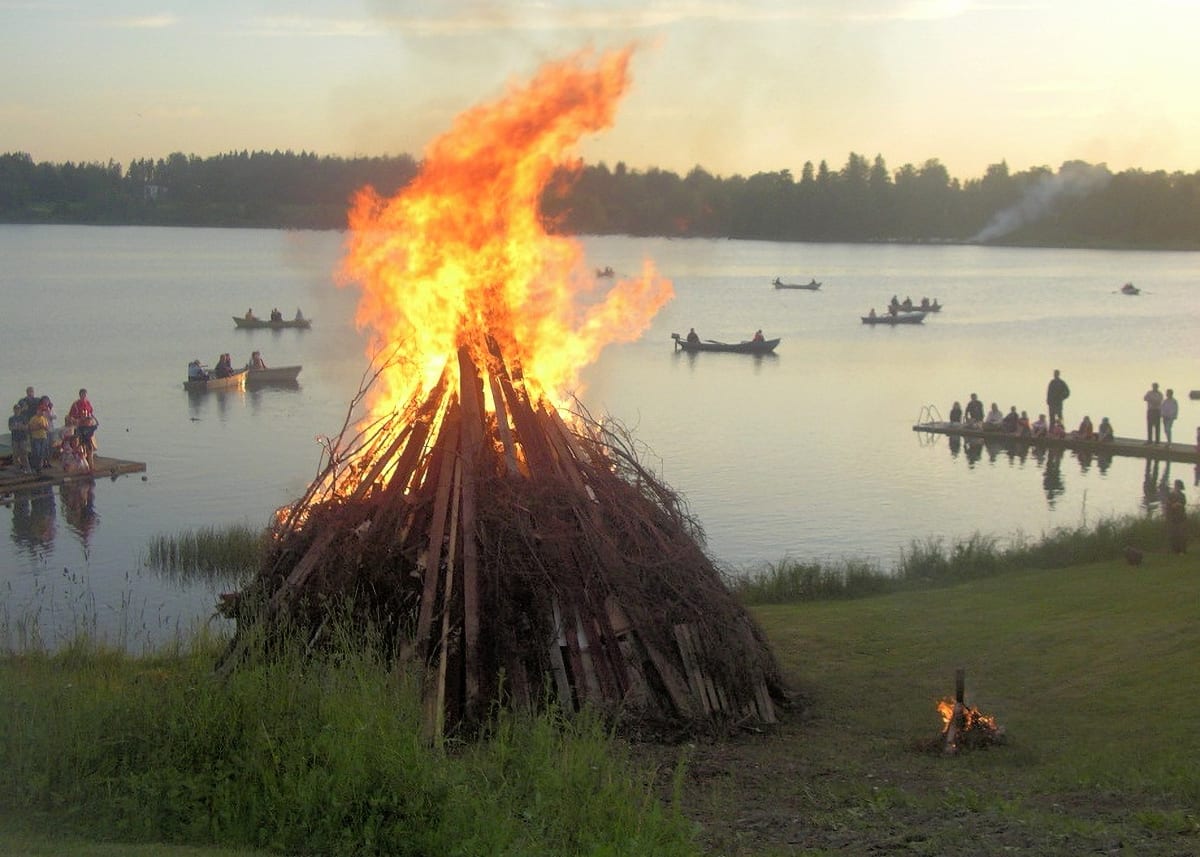In this detailed image set during the golden hour of sundown, vibrant orange flames leap from a towering bonfire composed of bundled branches and long strips of wood, positioned prominently on a grassy lakeside area. The bonfire, almost the height of a person, captivates the attention at the left of the center foreground. Surrounding the lake, children and adults gather on simple wooden piers on both the left and right sides, their silhouettes blurred into mere outlines against the evening light. In the background, a serene lake stretches out, dotted with about six small boats, each carrying two to three rowers, gliding peacefully across the reflective water. Above, a clear sky hovers over the distant treeline, completing the tranquil yet lively scene.